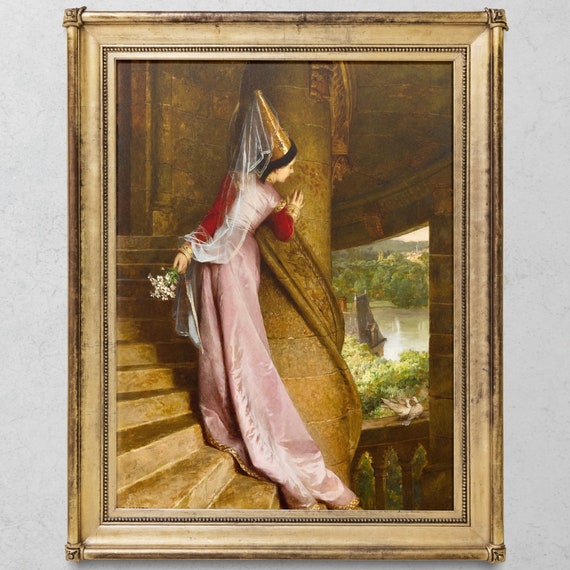A captivating old Victorian portrait hangs against a gray wall, encased in an ornate gold frame with darker gold borders, exuding a rustic and historic charm. The scene showcases the interior of what appears to be a grand castle. A spiral staircase, seemingly constructed from gold, wraps around a central column, guiding the viewer's eye towards a lady ascending the steps. She wears a flowing pink gown with burgundy sleeves and a gold, pointed hat that resembles a dunce cap. Her black hair cascades down as she delicately balances with her right hand on the golden pillar, while her left hand gently holds a small bouquet of white daisies. Through an open-air window adjacent to the staircase, two birds nestle on the sill, emboldened by the picturesque view outside—a serene lake or pond surrounded by trees with a ship afloat on its tranquil waters. This vintage artwork is both intricate and nostalgic, further accentuated by the gold-toned elements that dominate the portrait, contributing to its antique and rustic appearance.